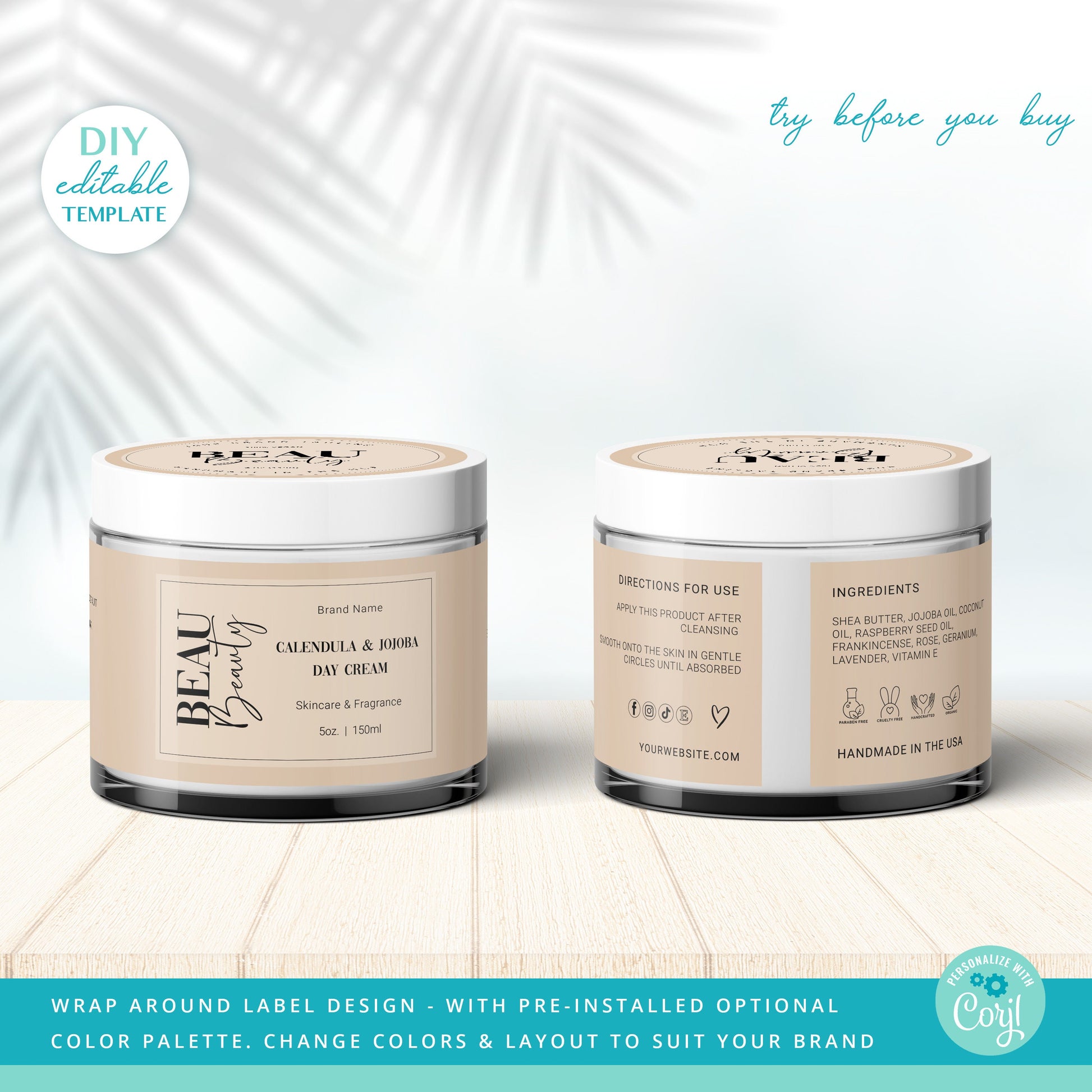The image in question displays two roundish canisters of skincare product, set against a white backdrop that includes a faint silhouette of palm tree leaves. Both containers are shown from different angles: the one on the left reveals the front label, and the one on the right displays the back with product details and ingredients. Each canister, made of a white cylinder with a twist top, features a brown label that reads "Bew Beauty Calendula and Jojoba Day Cream Skincare and Fragrance 5oz 150ml." The containers rest on a very light wood surface, and additional text elements enhance the visual presentation. In the top left corner, there is a sign that says "DIY Editable Template," while the top right corner reads "Try Before You Buy" in light blue or green lettering. The bottom part of the image includes a blue box with the words "Wrap Around Label Design with Pre-Installed Optional Color Palette. Change colors and layout to suit your brand." Lastly, the bottom right corner carries the phrase "Personalize with Courage."